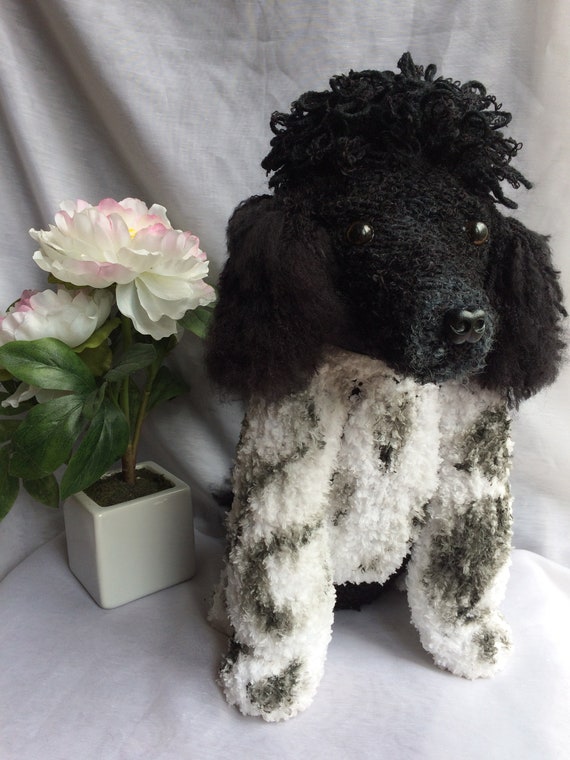The image showcases a meticulously knitted, life-size rendition of a poodle, featuring solid black curly afro-like hair and shiny brown eyes. The poodle wears a fluffy white sweater adorned with black splotches of amorphous shapes, covering its body down to the paws and midsection. The dog sits gracefully in front of a grey linen curtain. Positioned next to the poodle is a cubic white flowerpot containing a plant with a mix of pink-tinted white flowers and large green leaves. The overall scene combines a detailed, artistic representation of the poodle with a natural floral element.